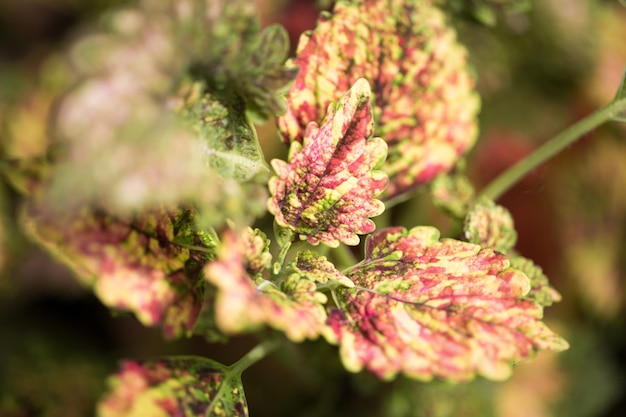This close-up photograph captures the leafy tip of a plant stem or branch from an overhead perspective. The image centers on a ring of variegated leaves that are arranged around the center stalk. These leaves are slightly rounded triangular or spade-shaped, exhibiting smooth, serrated edges with rounded lobes. Their coloration is a blend of green with striking ivory and pale red or pink hues. The stem extends off to the right and is slightly out of focus, blending into a background comprised of similarly blurred foliage in complementary shades of green, pink, and ivory. The warm tones and varied colors give a vivid, nature-rich feel to the scene.